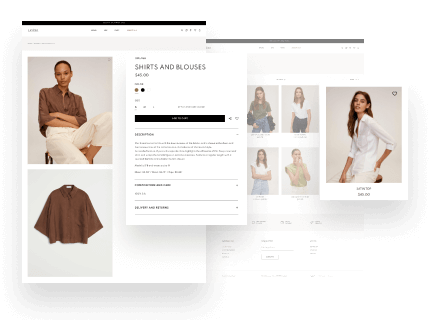This advertisement showcases a women's clothing website. The overall background is white, and the text is in black font. The ad features two main images: one arranged vertically, and the other horizontally, which slightly overlaps like a popup offering additional information about the site.

On the left side of the advertisement, there's a poised Black woman with short hair. She is dressed in a stylish brown button-down shirt with long sleeves and a flowy, patterned fabric. The shirt is paired with white pants. Beneath her image, the shirt is displayed separately, giving a clearer view of its design and texture.

The right side of the popup ad features a woman in a pristine white jumpsuit. She has darkish skin and brown hair, hinting at possible Hispanic heritage. Adjacent to her, four smaller images are arranged in a rectangular grid format, each showcasing her in different outfits, although the images are slightly grayed out. To the left of her, the text reads "Shirts and Blouses," followed by an “Add to Cart” button. Below these elements, there's additional information about the clothing, though it is too small to read from the screenshot provided. 

Overall, this advertisement effectively highlights the website's range of elegant and diverse women's clothing.